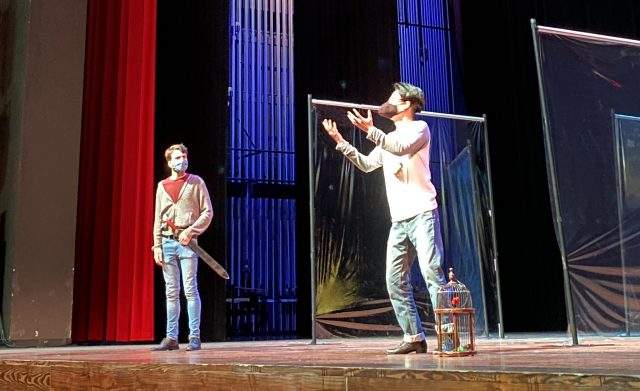The image depicts a stage performance featuring two men. The horizontally aligned rectangular photograph showcases a wooden stage floor with a small birdcage containing what seems to be a red bird positioned near the center stage. To the right, a man stands with his arms bent and palms facing upward, as if pleading. He is dressed in a long-sleeved light-colored shirt, rolled-up jeans, and a brown medical mask over his ears. To the left, another man stands facing forward, donning a tan shirt with a red T-shirt underneath, blue jeans, and a blue medical mask. He holds a sheathed sword with a hand placed on its hilt. The background features towering red curtains and tall, clear rectangular windows or plastic partitions, bathed in ambient blue light, suggesting an older theatrical setting possibly adapted for COVID-19 precautions.